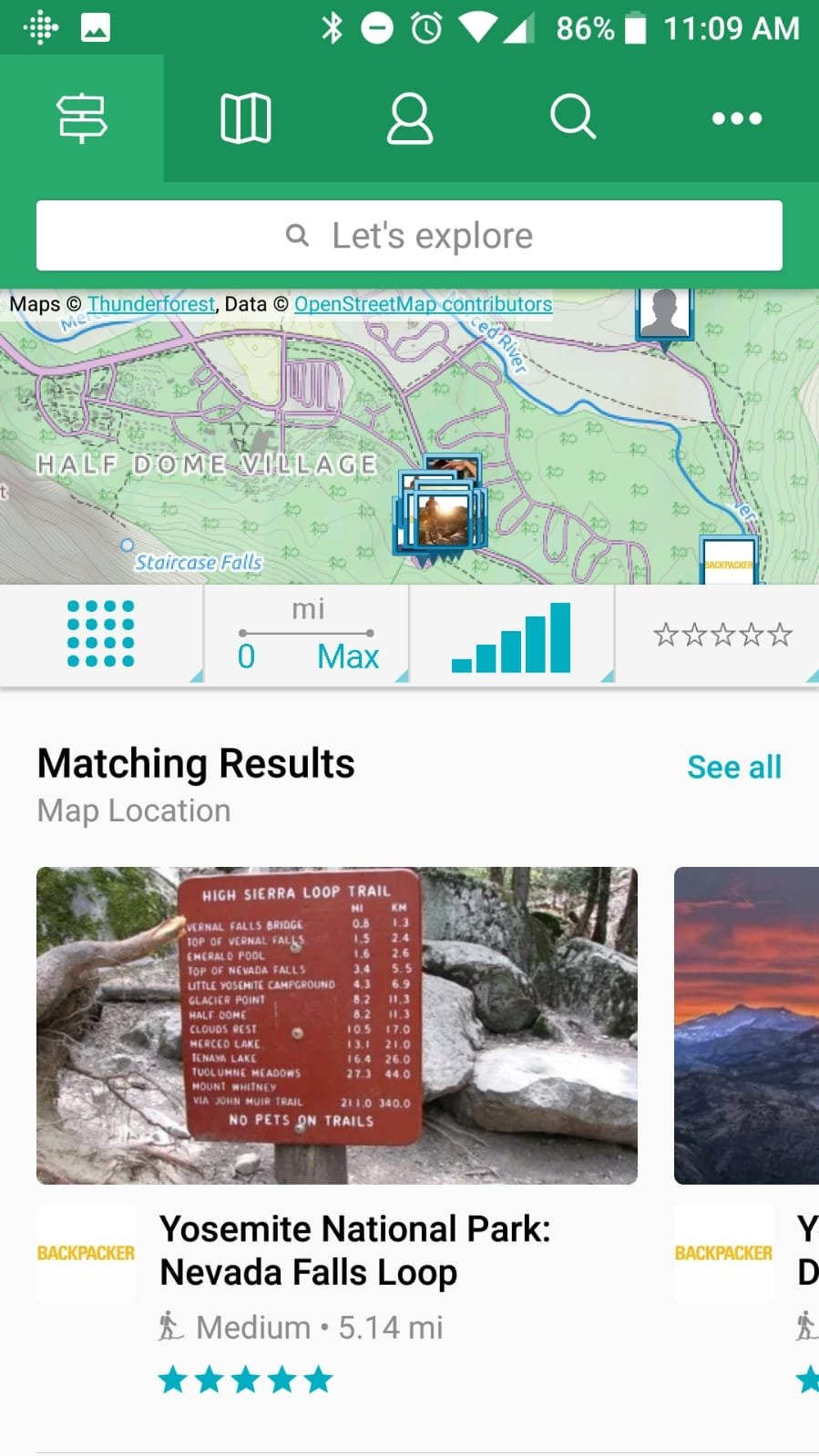An image captured from an old Android phone interface displays what appears to be a screenshot of either the Google Play Store or Google Maps, featuring a dated and simplistic design. The background of the interface is predominantly white. 

At the very top right-hand corner, several status indicators are visible: the time reads 11:09 AM, the battery is 86% charged, Do Not Disturb mode is activated, Bluetooth is on, and symbols for Wi-Fi connectivity, cellular signal strength, and an alarm or timer are displayed. 

Beneath these status icons, a search bar is prominently positioned bearing the text, "Let's Explore." Directly below the search bar is a map showcasing user locations, with one prominently marked as Half Dome Village. The top left-hand corner of the map includes a small legend that reads, "Maps Copyrighted, Thunder Forest."

At the bottom of the screen, matching results are listed, with the primary one being Yosemite National Park, Nevada Falls Loop, which boasts a 5-star rating. Another location is partially visible to the right but is cut off, making it unreadable.